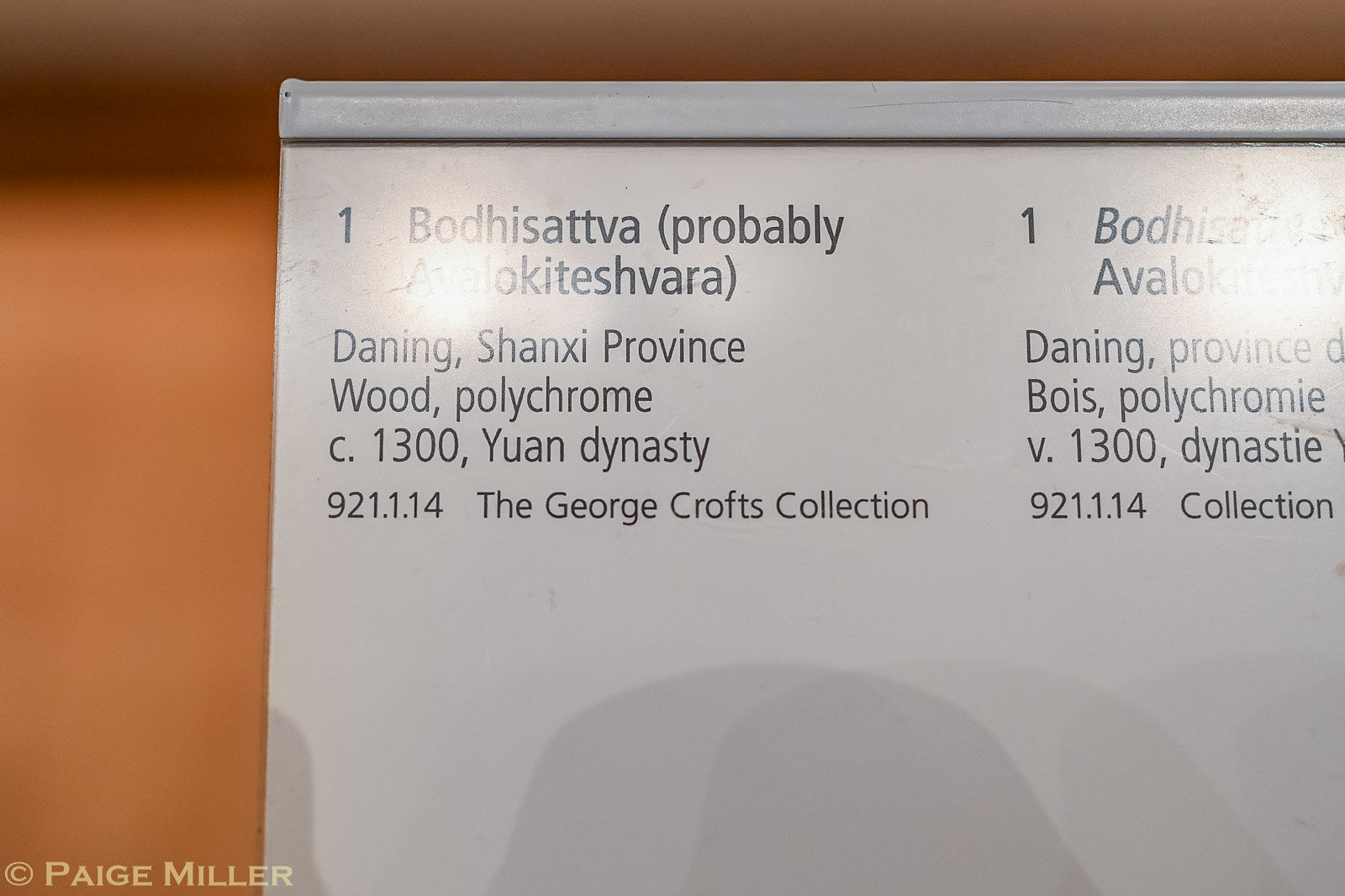This color photograph, set in landscape orientation, captures a detailed image of a descriptive placard likely seen in a museum setting. The placard, primarily white with gray text, is shown against a blurred light brown background. The background fills the left fourth of the image, while the zoomed-in placard occupies the right three-fourths. The text on the placard provides information about an artifact: it reads "Bodhisattva (probably Avalokiteshvara)," followed by "Daning, Shanxi Province," and describes the material as "Wood, Polychrome," dating back to "C.1300, Yuan Dynasty." Below these details, it lists a serial number "921.1.14" and attributes the item to "the George Crofts Collection." The setting and style of the photograph suggest a museum environment, and the placard appears to describe an artifact above it that is not shown in this image. The entire composition is in a realistic photographic style, with a clear emphasis on the placard's detailed information.